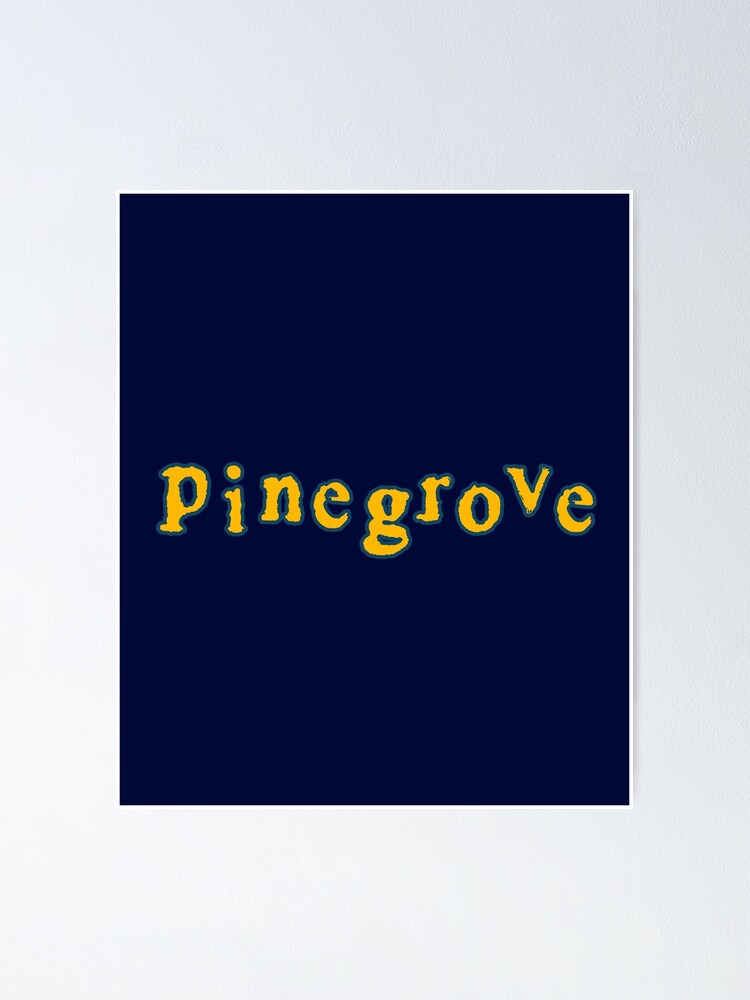This image features an advertisement for a poster or art print set against a light gray to medium white-gray gradient wall, likely CGI-generated. The central focus is a vertically oriented, navy blue rectangle framed by a delicate white border. At the heart of this dark navy field, yellow distressed serif letters spell out "Pine Grove," each uniquely offset, giving them an uneven, bouncing appearance. The letters vary slightly in size and height, adding to the hand-drawn aesthetic, and are subtly outlined in a very dark teal, nearly blending into the navy backdrop. This playful, yet carefully designed composition stands out prominently against the understated background.